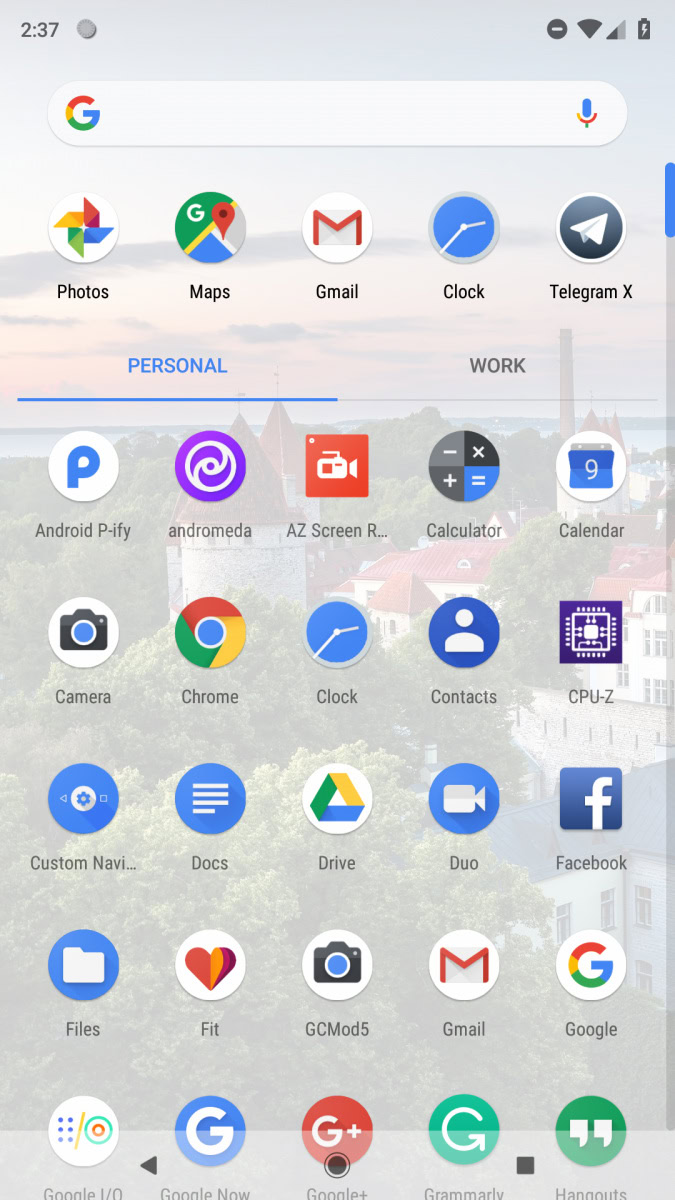Screenshot of a smartphone home screen displaying a variety of apps organized in rows. At the top, there's a Google search bar followed by an array of Google apps, including Google Photos, Google Maps, Gmail, and Google Clock. Telegram X is also present, represented by an airplane icon. Below these, the screen features a text notification badge reading "Android P update available," alongside a purple icon for Andromedia.

Other app icons include AZ Screen Recorder (depicted by a red box with a camera symbol), Calculator (a circle with mathematical symbols), and Calendar (a circle with a line). The bottom row includes essential apps like the Camera, Chrome, Clock, Contacts, and a square icon for CPU monitoring. There are further apps such as Custom Navigation, Google Docs, Google Drive, Google Duo, Facebook, Files, Google Fit, a secondary Camera app labeled GC Mod 5, Gmail, the primary Google app, Grammarly, Google Plus, Google Now, and Hangouts.

The home screen boasts a background image of a picturesque village, possibly located overseas, with charming architecture and lush greenery, providing a serene and captivating backdrop.